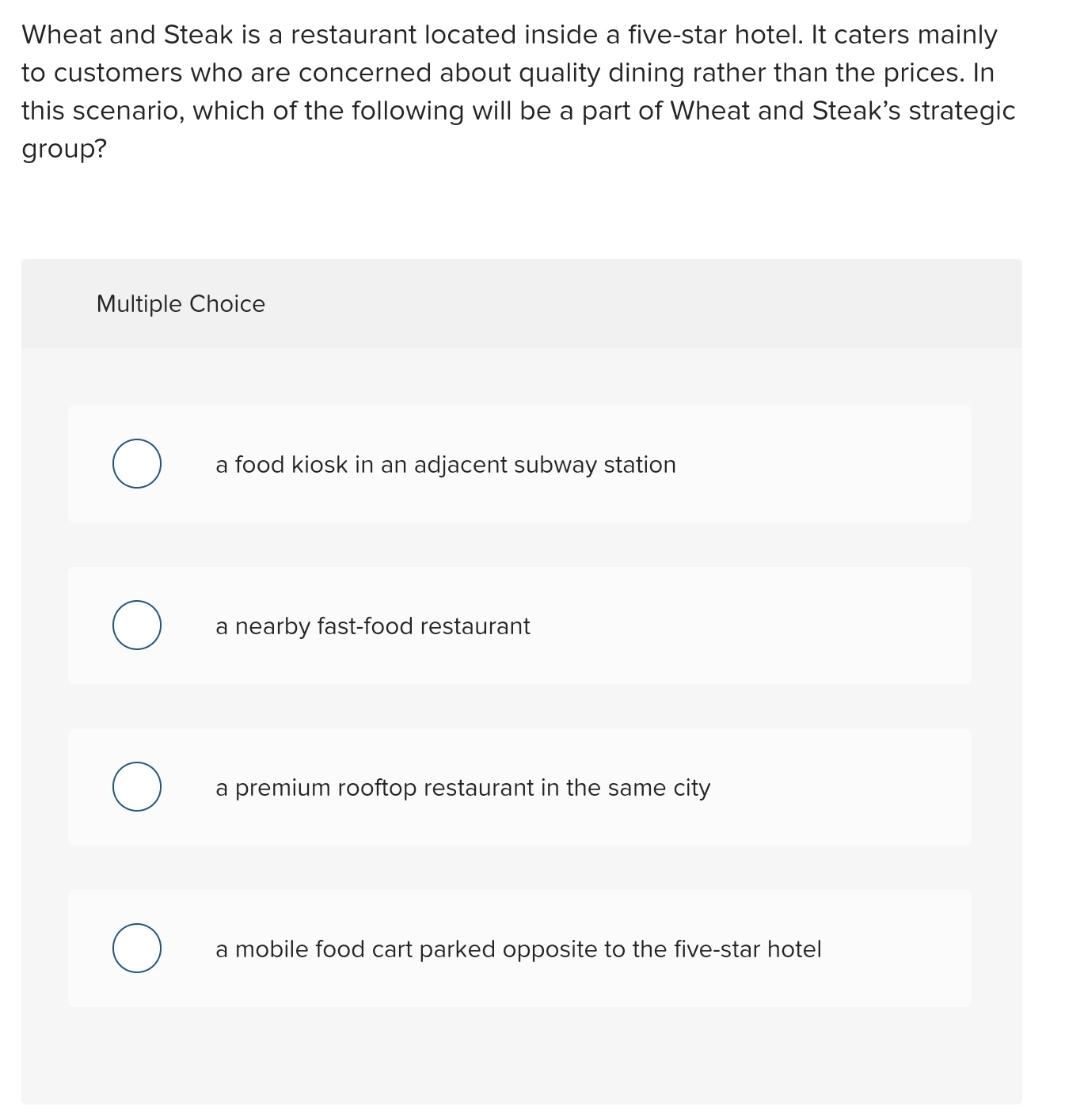The image depicts a survey set against a clean, white background. At the top of the image, there is a question in black text, which reads: "WeInSteak is a restaurant located inside a five-star hotel. It caters mainly to customers who are concerned about quality dining rather than prices. In this scenario, which of the following will be part of WeInSteak's strategic group?" Beneath this question, there is a very light gray rectangular section containing the multiple-choice options. Each option is presented in its own white rectangle, with a corresponding circle to the left for selection. The choices listed are:

1. A food kiosk in a subway station
2. A nearby fast food restaurant
3. A premium rooftop restaurant in the same city
4. A mobile food cart parked opposite the five-star hotel